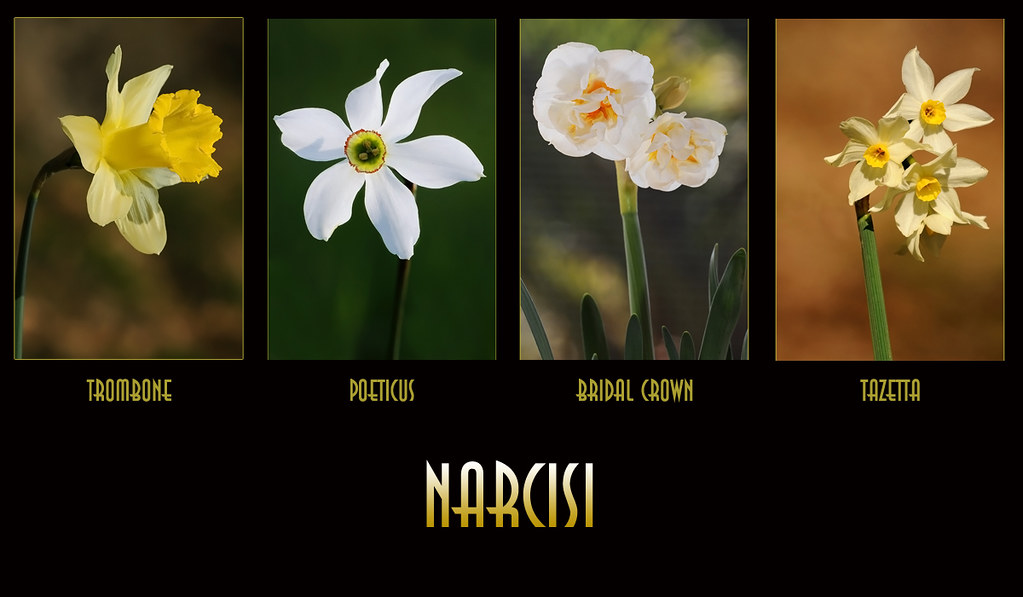The image features a detailed, professional-looking assortment of four types of Narcissus flowers, displayed against a black background in a horizontal layout. From left to right, the first flower is labeled "Trombone" and boasts petals of two shades of yellow, with a distinctive protruding section resembling a trombone's pipe. Adjacent to it, the second flower is labeled "Poeticus" and showcases six pristine white petals encircling a yellow center. The third flower, named "Bridal Crown," exhibits a fuller arrangement of white petals with a creamy undertone. The last flower on the right is called "Tazetta" and uniquely displays a cluster of three white flowers with star-shaped appearances. Below each flower, their respective names are labeled, with the word "Narcissi" written at the very bottom in a green-to-white gradient text, indicating the variety within the Narcissus family.